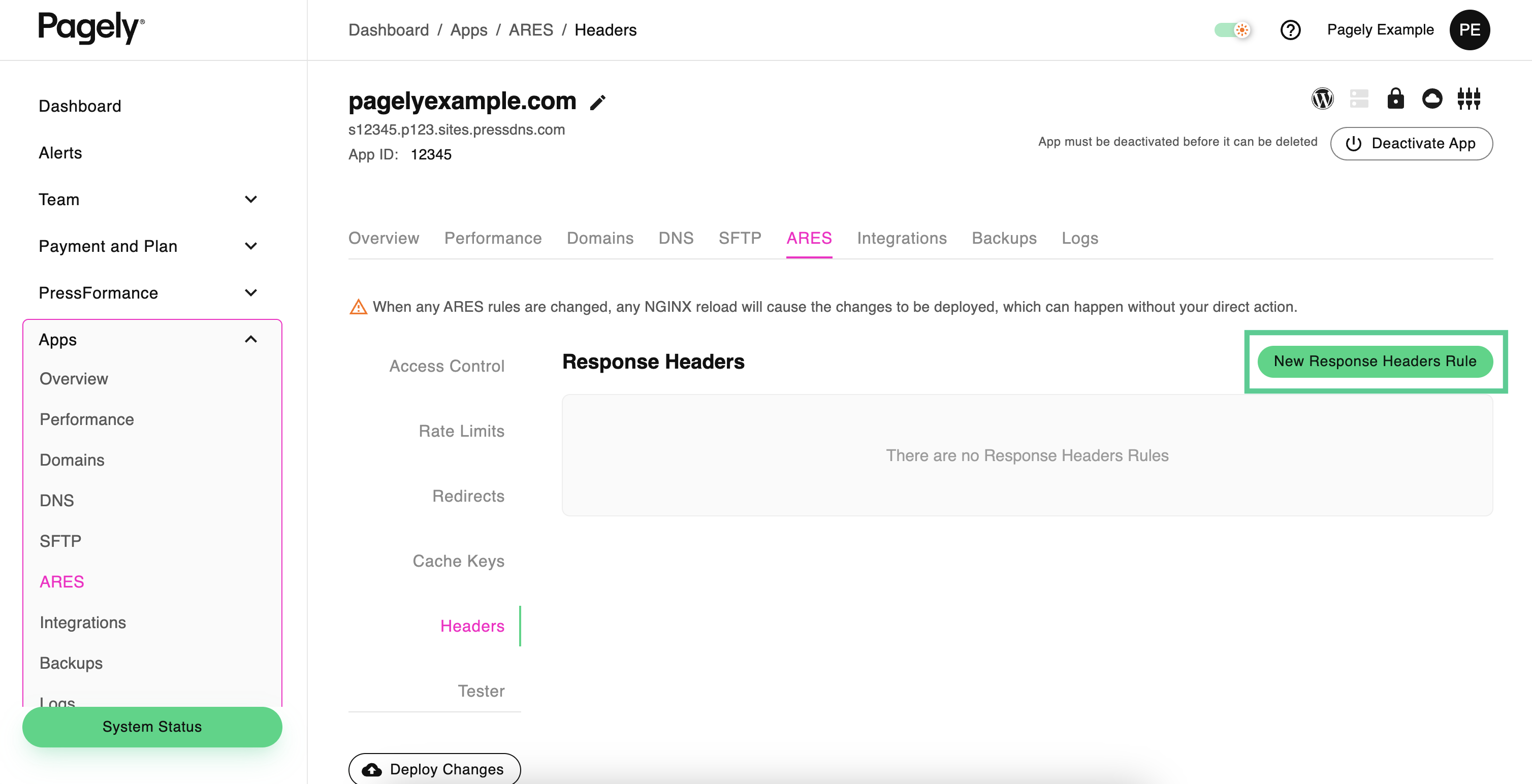The image displays a detailed interface from the Pagely dashboard. In the upper left corner, "Pagely" is prominently written in black text, followed by a series of categories in black: Dashboard, Alerts, Team, Payment and Plan, Press, and Formats. Below these, inside a pink square, is the word "Apps." Further down the list, additional categories are noted: Overview, Performance, Domains, DNS, SFTP, and ARES, which is emphasized in bold pink text. The list concludes with Integrations and Backups.

To the right of this, "PagelyExample.com" is displayed, and an image of a black pencil or another writing utensil is present. Here, the same categories appear but are arranged horizontally, with "ARES" again highlighted in bold pink and underlined in pink.

On the far right, there is a green oval shape with a horizontal orientation, outlined by a green-lined rectangle. Inside this oval, it reads: "New Response, Headers, Roll." In the upper right corner of the image, "PagelyExample" is written with a black circle to its right. This detailed layout highlights the organized structure and key features available within the Pagely dashboard interface.